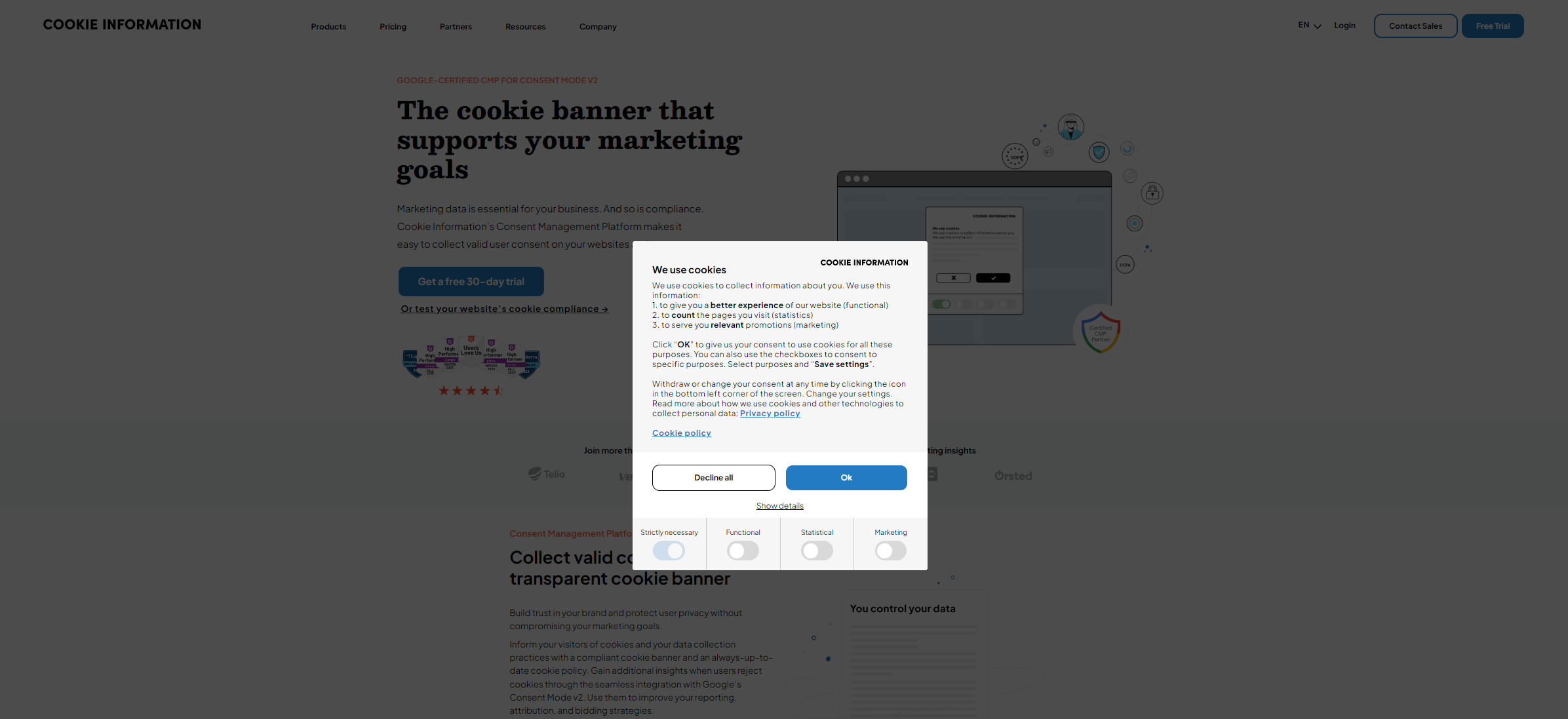The image is a screenshot from a website featuring a prominently displayed white pop-up box that obscures the grayed-out background. The backdrop includes a webpage layout with navigational elements such as "Products," "Pricing," "Partners," "Resources," and "Company" listed across the top menu. On the far right, there are options to change the language ("EN" for English) via a dropdown menu, log in, contact sales, and initiate a free trial.

In the grayed-out background, there is text discussing cookie information, while centrally positioned on the page in red font is the headline "Google Certified CMP for Consent Mode Volume 2." Below this, in black font, is the subheading "The cookie banner that supports your marketing goals," followed by a brief descriptive paragraph.

The white pop-up box in the center provides detailed information about cookie usage, including the purpose of functional cookies, statistical tracking of page visits, and serving relevant promotions. At the bottom of this pop-up, users are given two options: "Decline All" or "OK."